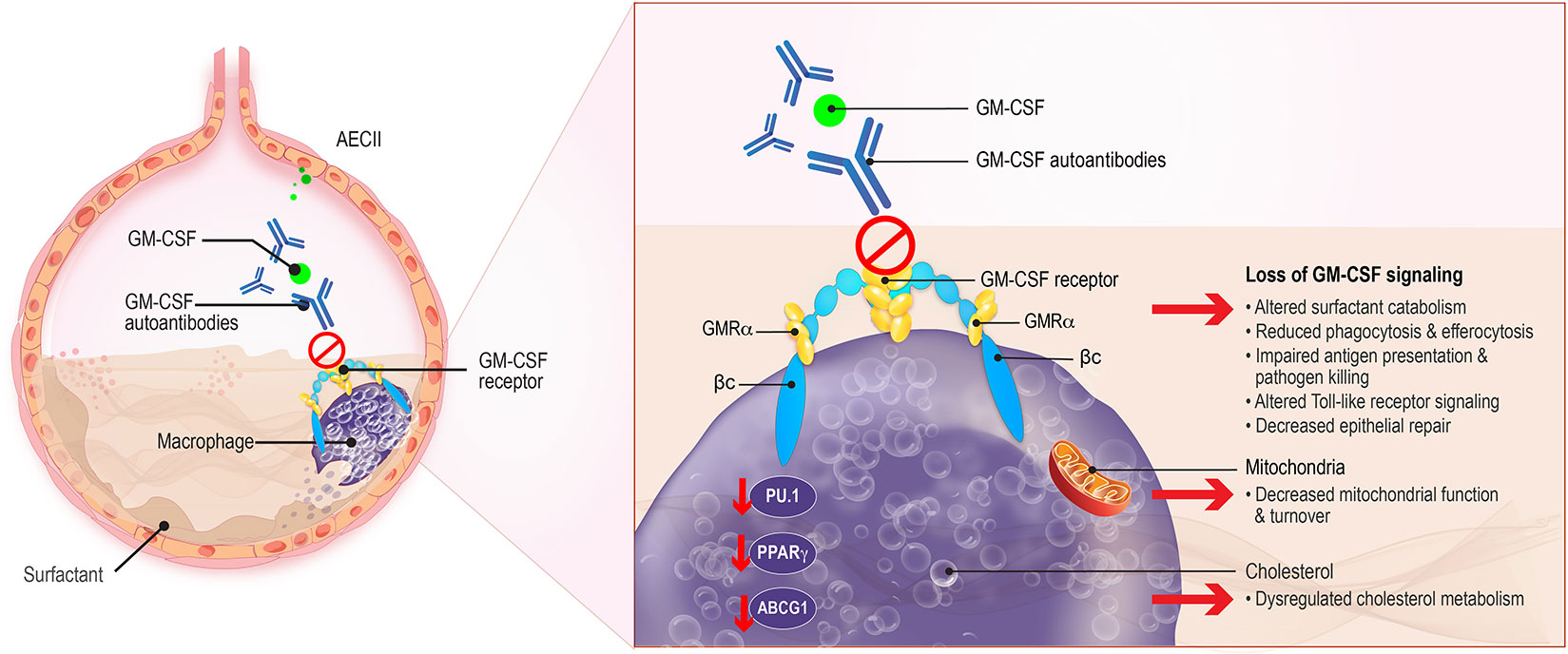This is a detailed medical diagram likely taken from a medical textbook, depicting a purple, round cell, identified as a macrophage. The macrophage, prominently labeled, features a variety of specific components marked by descriptors. The cell includes several key parts such as GM-CSF (Granulocyte-Macrophage Colony-Stimulating Factor) autoantibodies, mitochondria, and cholesterol, all highlighted with pointers and text. A focal point of the diagram is the loss of GM-CSF signaling, prominently displayed in a separate, enlarged box to the right of the main cell image. This box outlines various conditions associated with the loss of GM-CSF signaling including reduced phagocytosis and electrogenesis, impaired antigen presentation and pathogen killing, and altered toll-like receptor signaling, marked with red arrows. The macrophage also contains small white bubbles representing different cellular components and receptors. The overall diagram meticulously details the dysregulation and various cellular irregularities within the macrophage.